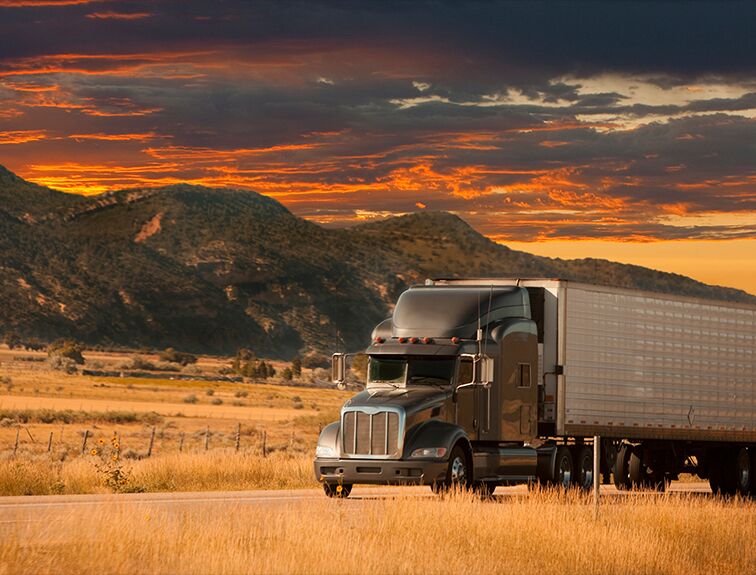The photograph captures a scenic evening scene featuring an 18-wheeler semi-truck traveling down a flat, old country road. The truck itself has a gray cab and a white container trailer. The road is bordered by brown grass and weeds, with a barbed wire fence and wooden fence post visible on one side. In the foreground, the land appears dry and tan, possibly resembling hay or straw fields. The background reveals rolling hills or tall mountains, with deeper green vegetation at the base, gradually blending into a hilly terrain. Above this landscape, the sky manifests the onset of sunset, featuring a gradient of darker blue at the top, transitioning through striking hues of orange, yellow, and purple streaks. Scattered white clouds add texture to the vivid sky, which completes the captivating backdrop for the semi-truck making its journey.